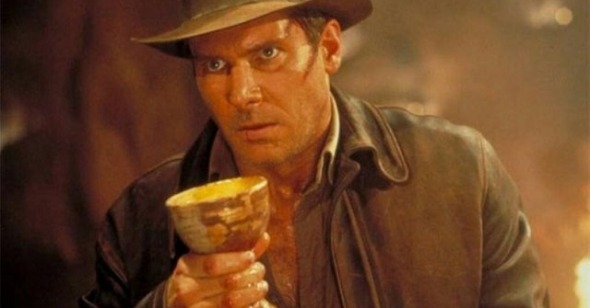This image is a detailed drawing capturing Harrison Ford as Indiana Jones from "Indiana Jones and the Last Crusade," in which he is holding the Holy Grail. Indiana Jones, with his trademark light brown leather hat and medium brown leather jacket, faces the camera but gazes intently to the right. His grayish brown shirt is partially unbuttoned, revealing a bit of his chest, and both his face and hands appear sweaty, emphasizing the intensity of the scene. The rough, weathered chalice clutched in his right hand is central to the image. His stern, concentrated expression, together with piercing blue eyes, adds to the dramatic ambiance. The background evokes the iconic yellow or gold hue typical of the film’s underground cave settings with a torchlight subtly illuminating the surroundings. A faint injury line can be seen on the right side of his face, hinting at recent action and danger.